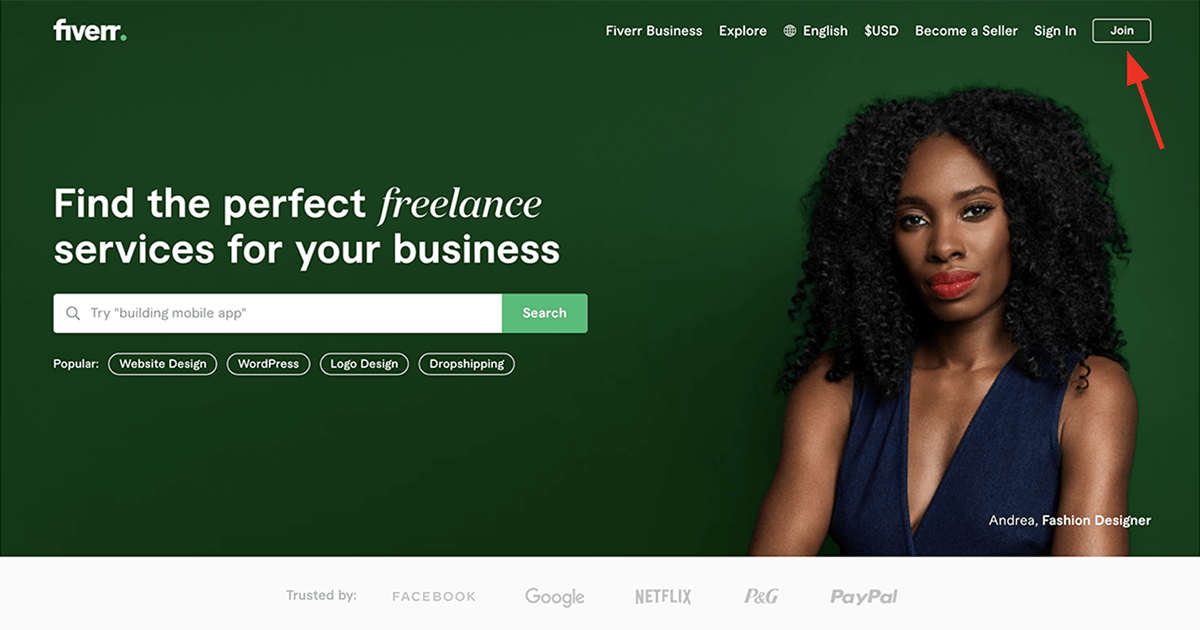This screenshot from the Fiverr website showcases various features and elements designed to assist users in finding freelance services for their business needs. In the top left corner, the word "Fiverr" is displayed in all lowercase letters. Moving across the top of the page to the right corner, the header reads "Fiverr Business Explorer" beside an icon of a globe. Further along the top, it shows language, currency options (indicated by "English, USD"), and links for "Become a Seller," "Sign In," and a highlighted "Join" button bordered in white, pointed to by a red arrow.

Dominating the right side of the screenshot is an image of an African American woman with long, curly hair cascading slightly below her shoulders. She is gazing into the camera with a subtle smile, dressed in a sleeveless black dress that reveals her arms up to just above the elbows, making it a headshot that includes her shoulders and upper arms. Overlaying this image on the lower right side, in white text, is the caption "Andrea, Fashion Designer."

On the left side of the screenshot, the largest text on the page reads, "Find the perfect freelance services for your business" in white. The word "freelance" is in a distinctive script that makes it stand out from the rest of the text. Beneath this headline is a search bar with the placeholder text suggesting "try 'building mobile app'" and a green "Search" button to its right. Below the search bar, it lists popular services including "Website Design," "WordPress," "Logo Design," and "Drop Shipping."